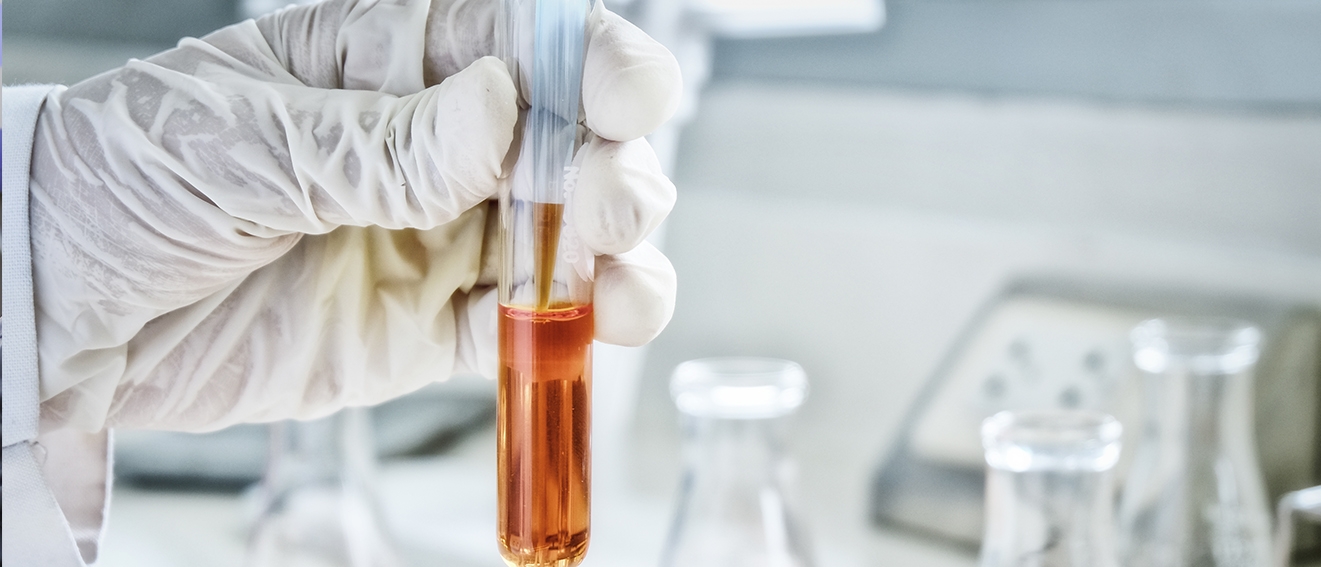A horizontal color photograph captures a scientist in a white lab coat and white latex gloves, focusing intently on his task in a laboratory setting. Although the scientist himself is mostly obscured, his left hand is prominently featured, holding a slender test tube. The test tube contains an amber-colored, possibly orange or golden brown liquid that fills about one-third of the tube. In his other hand, partially visible, the scientist appears to be using a syringe to either extract or add the liquid. The background is blurred, revealing various pieces of scientific equipment, empty tubes, beakers, and grayish walls, ensuring that the viewer's attention remains on the meticulous handling of the test tube and its contents.